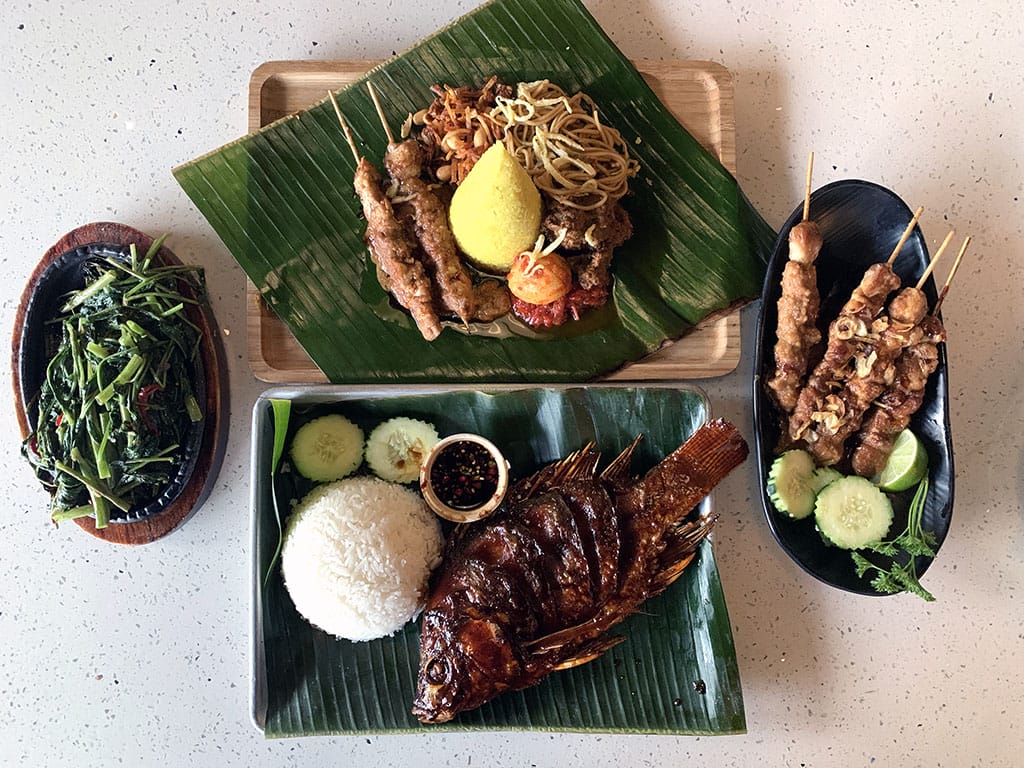In this photograph of an Asian-inspired meal set indoors, there are four distinct dishes artfully arranged on a white speckled surface. The centerpiece includes a whole fried fish with a rich red sauce, accompanied by a mound of white rice, cucumber slices, and a dark soy dipping sauce in a small white bowl. Adjacent to this is a rectangular wooden tray topped with a green leaf, possibly banana or seaweed, featuring skewers of cylindrical meat, a cluster of noodles, and colorful vegetables, including yellow, orange, and red spherical items. To the left is an ovular wooden trivet holding a black plate filled with what appears to be grilled or stir-fried watercress or similar greens. On the right, a black oval bowl contains four skewers of meat, garnished with cucumber slices, a lime wedge, and sprigs of parsley. Each dish is presented elegantly on banana leaves, adding a rustic and authentic touch to the vibrant and appetizing spread.